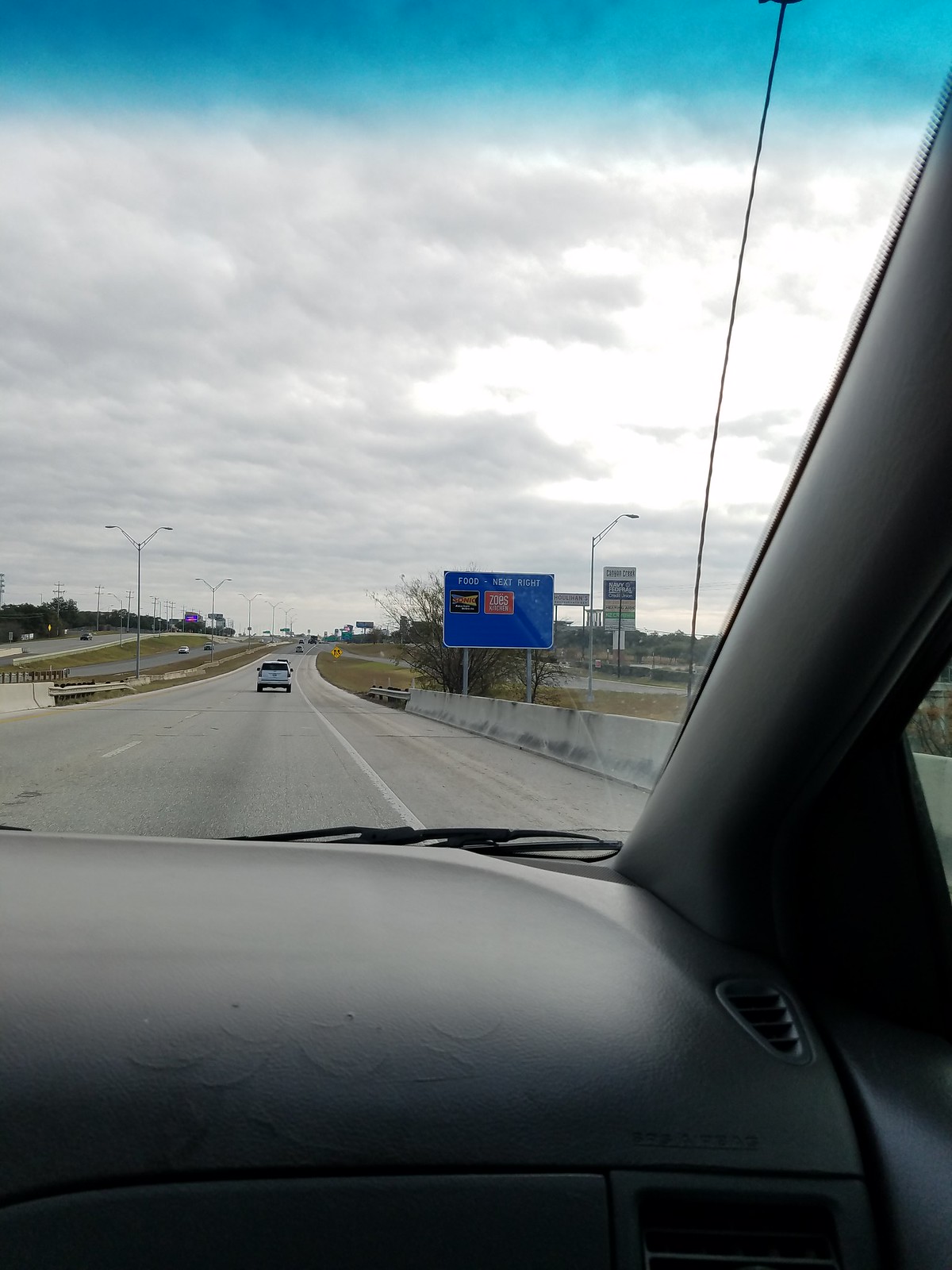Photographed from the passenger seat of a car, this image captures a blue sign situated on the right side of a highway. The dashboard, heater vent, part of the windshield wiper, and the window, along with the car's antenna, are visible within the vehicle. Outside, the blue sign is supported by two gray posts and features multiple elements: a yellow and black badge with "Sonic" written in red letters, followed by another sign indicating "Zoe's Kitchen" in white letters against a red background. Adjacent to this, a taller sign displays several pieces of information. A tree or bush stands behind the blue sign, and a concrete half-wall barrier borders the right side of the frame. In the lane ahead, a white SUV with tinted windows is visible, along with street lights. The scene is set under a cloudy sky, and another highway can be seen across a gully to the left, with a few cars on it.